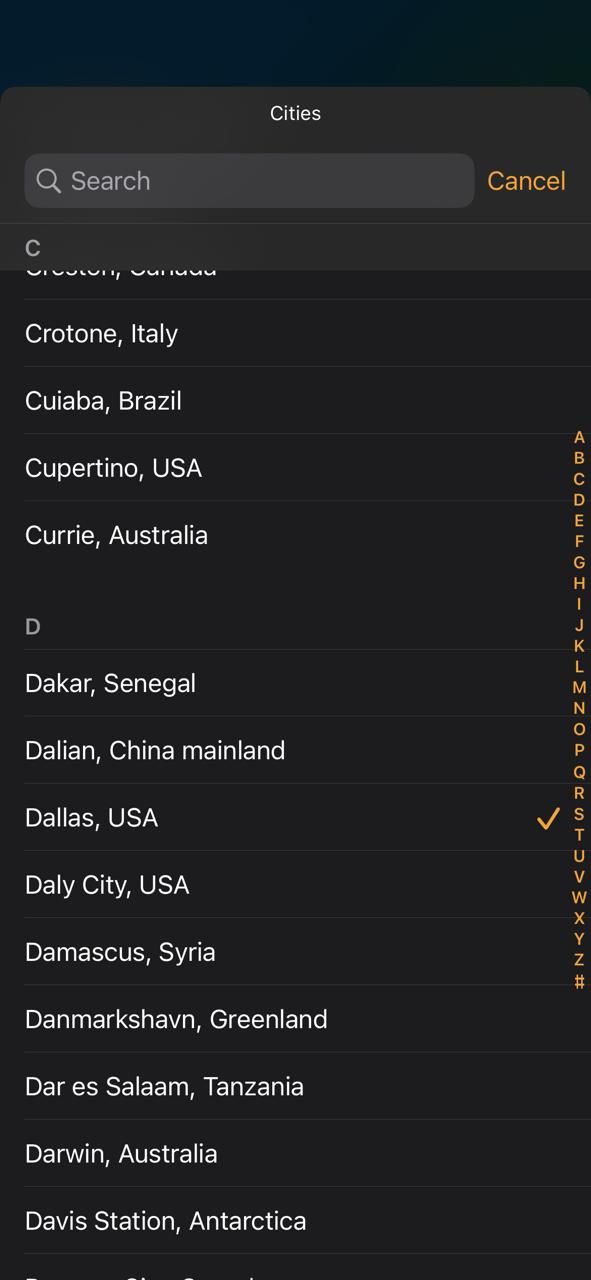This screenshot depicts a smartphone interface where a user is searching for cities, possibly for weather information. The screen displays a pop-up with the header "Cities," a search bar to hasten selections, and a "Cancel" button to exit the pop-up. The list begins with cities whose names start with 'C,' including Crotone in Italy, Cotone in the USA, Curie in Brazil, Curie in Australia, followed by cities starting with 'D,' such as Dakar in Senegal, Dalian in Mainland China, Dallas in the USA (already checkmarked), Daly City in the USA, Damascus in Syria, Denmark in Greenland, Dar es Salaam in Tanzania, Darwin in Australia, and Davis Station in Antarctica. An alphabetical navigation strip appears on the side for quicker access to cities by their initial letter. The checkmark next to Dallas, Texas indicates it is the selected city, suggesting Dallas was the intended search.